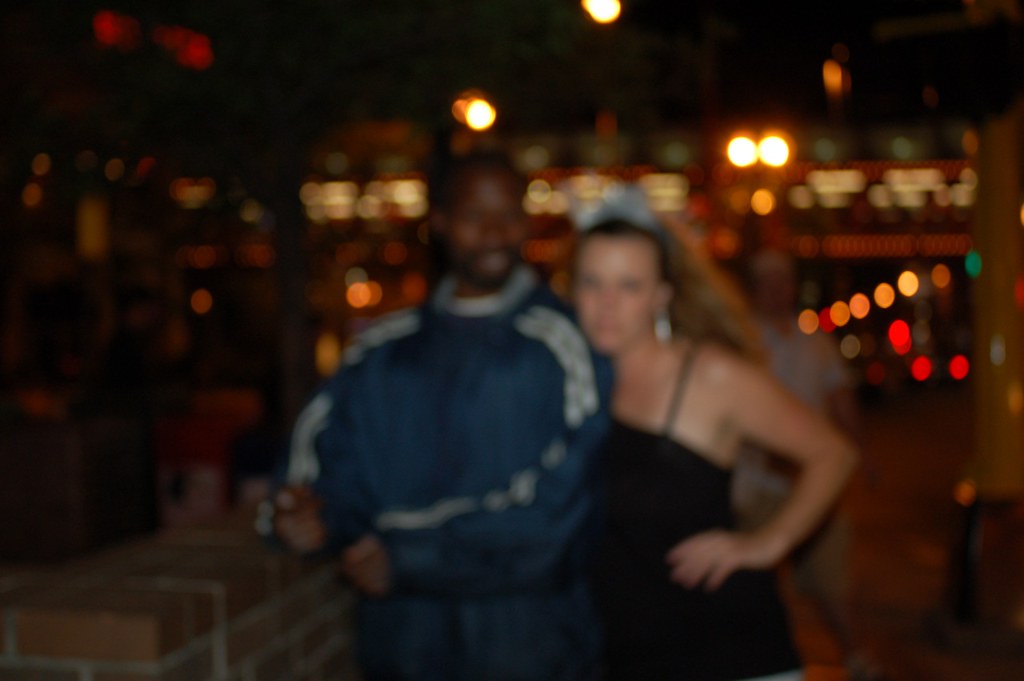The photograph is a horizontally-oriented, unfocused color image capturing a dimly-lit restaurant or bar ambiance. Dominated by warm colors, the background showcases a playful mix of orange, yellow, red, and green lights, creating a festive atmosphere. 

At the center stand a couple engaged in the moment. The man on the left dons a blue and silver windbreaker jacket, exuding a casual yet trendy vibe. Beside him is a woman in a strapless black dress, her hand confidently placed on her hip. Her outfit is accented by a possible crown atop her head and a long, elegant earring that gleams subtly in the lighting. 

The man's gaze is directed slightly past the woman's head towards the bottom right of the image, adding a layer of intrigue to the scene. In contrast, the woman faces forward, her direct gaze adding a touch of poise and confidence. The overall warm color palette and blurriness lend the photo a cozy yet mysterious feel, encapsulating the lively energy of the setting.